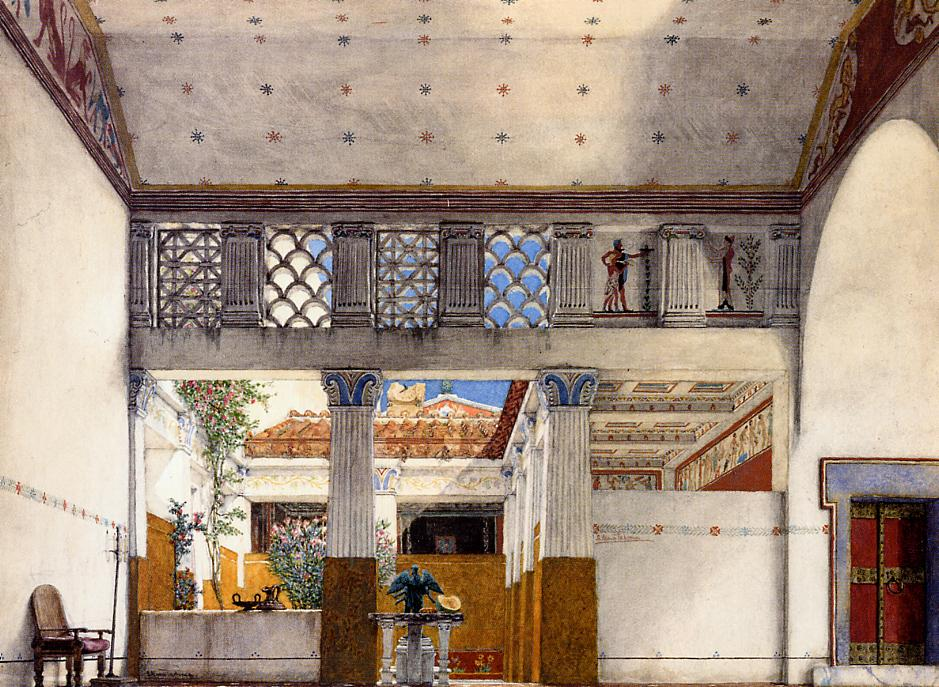The image, a vivid and colorful painting, appears to depict a Roman or Greek-style building, characterized by its insulate design with an internal courtyard. The setting is both indoor and outdoor, offering a seamless transition between the two through a wide opening that blends elements of the exterior with the interior. Dominating the foreground is the inside ceiling of the first room, adorned with a star pattern featuring touches of red and blue. Below this ceiling, four windows offer a view to the outside, framed by two prominent pillars.

Progressing into the scene, the repetition of these pillars guides the perspective through a courtyard filled with lush greenery, including shrubs and small trees. Centrally located within the courtyard is a birdbath, crowned with a statue of a bird. Whitewashed walls connect various sections of the structure, punctuated by strong right angles and colorful windows that add to the vibrant aesthetic.

To the left of the scene, a wooden chair is positioned against the wall in the first room, contributing to the image's serene atmosphere. On the right, a doorway punctuates the bottom corner of the room, suggesting further spaces to explore within the home. The other side of the courtyard reveals more of the building, its roof, and the blue sky beyond, encapsulating the serene and open nature of this meticulously detailed painting.